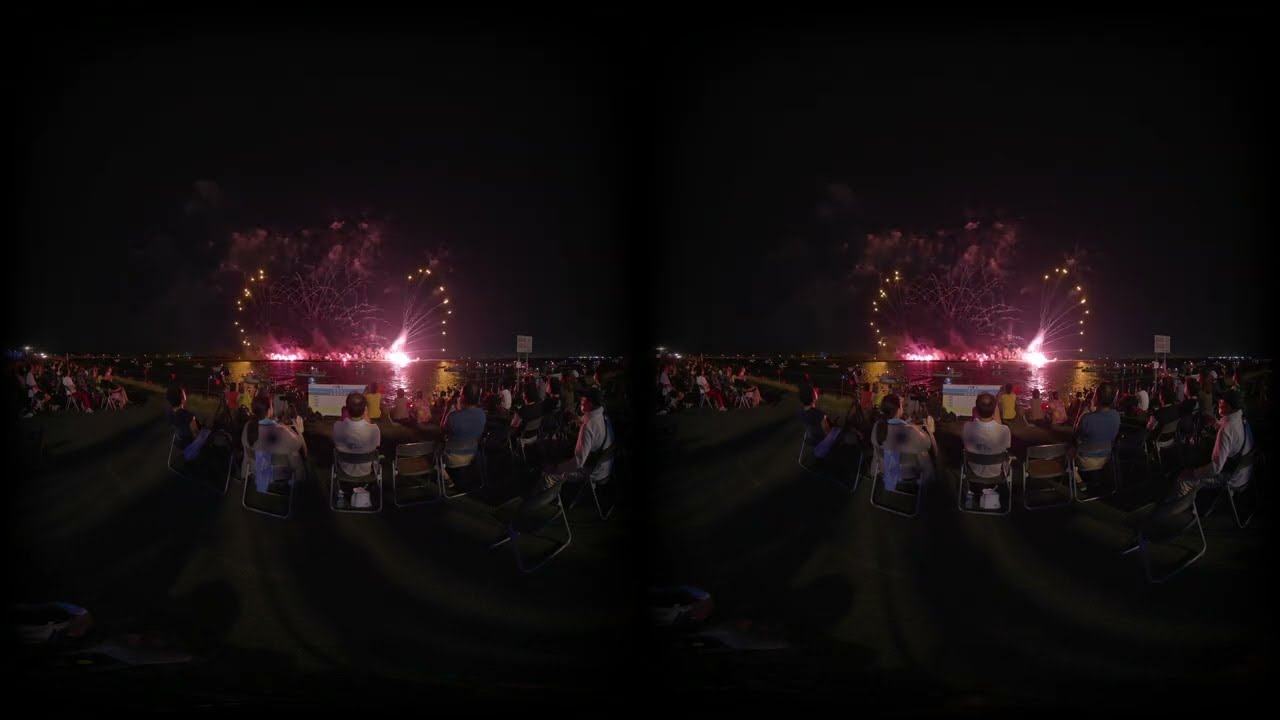The photograph captures a lively nighttime scene where a large crowd is gathered to enjoy a fireworks display by the water's edge. The sky is pitch black, illuminated by magenta and gold-tipped fireworks that fizzle and arc outward, reflecting beautifully on the water below. The crowd, sitting on an array of plastic and metal lawn chairs on a tan or grassy surface, is diverse, with many dressed in white, while some sport blue and red attire. The crowd spans across both the left and right sides of the image, with people intently watching the colorful spectacle. Among them, two individuals in grey attire are distinctly visible seated on light brown chairs. The image is available in a dual-frame format, where identical photographs are placed side-by-side, enhancing the sense of the event's scale and communal enjoyment.